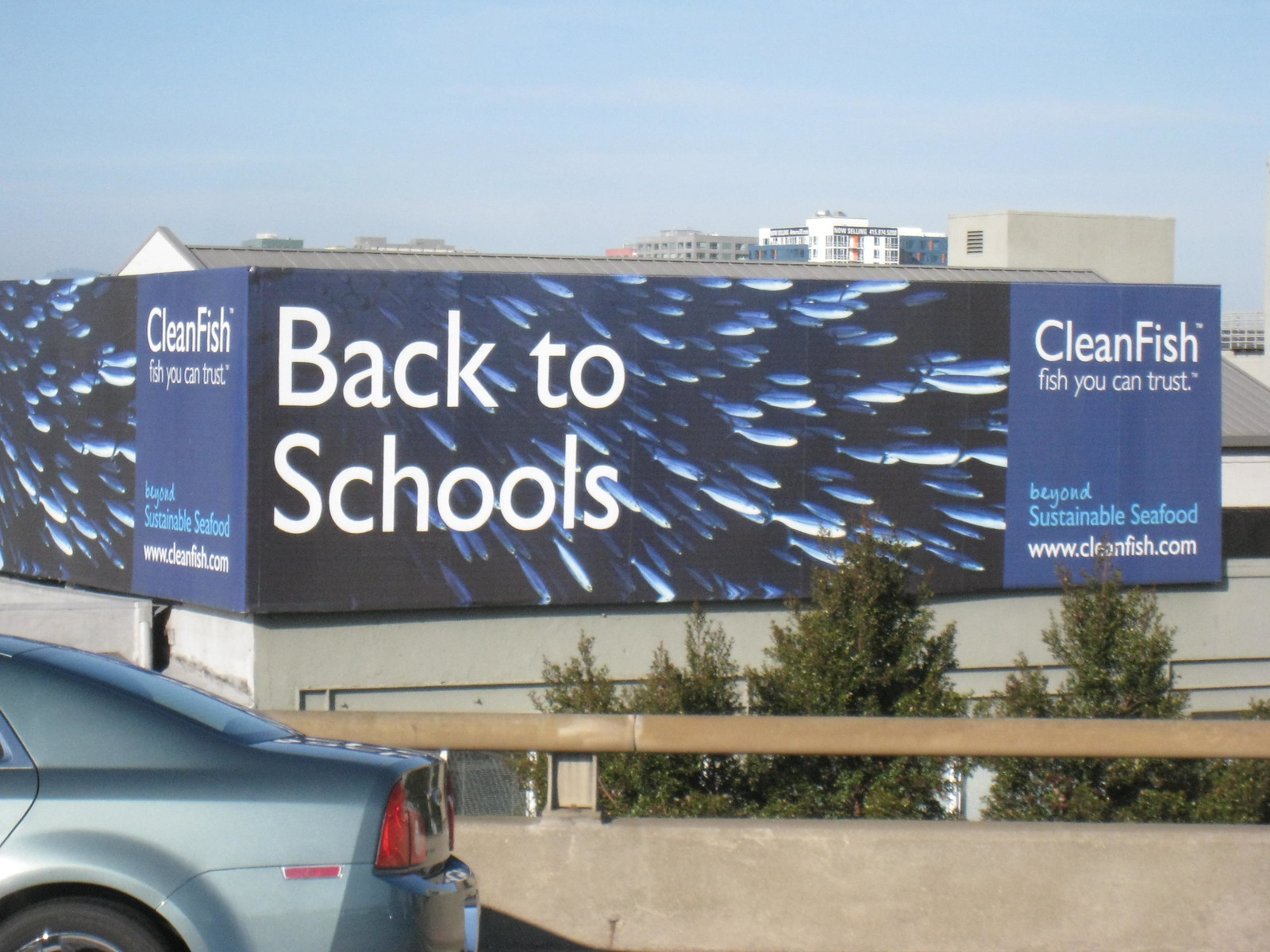The image features a building adorned with an advertisement that reads, "Back to School. CleanFish: Fish You Can Trust. Beyond Sustainable Seafood." The advertisement also includes a website address: www.cleanfish.com. The building, likely a supermarket, promotes sustainable seafood products. The setting is enhanced by a number of trees lining the side of the building in the foreground. A highway runs in front of the building, and a vehicle—possibly a Ford Focus or a Honda City—is captured just about to exit the frame on the left-hand side. The scene seems to be bathed in daylight, suggesting the photo was taken around 2 p.m.